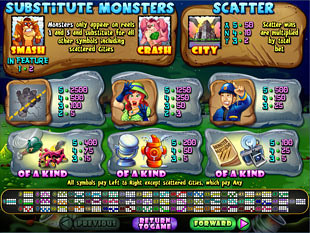The image is a screenshot of a busy-looking video game interface. The top header features the text "Substitute Monsters" in light blue, capital letters. Adjacent to this, on the upper right, is the word "Scatter", also in capital letters. Below the "Substitute Monsters" section, there are two character portraits: the one on the left is brown, the one on the right is pink, labeled "Smash" and "Crash" respectively. In the "Scatter" section beneath, there's a triangular-shaped portrait labeled "City." Underneath these categories, there are six gray rectangles arranged in a grid with two character portraits and four items, likely depicting various tools or equipment. The bottom section of the screenshot shows text including "Return to Game" and "Forward," along with numerous unreadable numbers and words, which are presumably stats and options related to the gameplay.